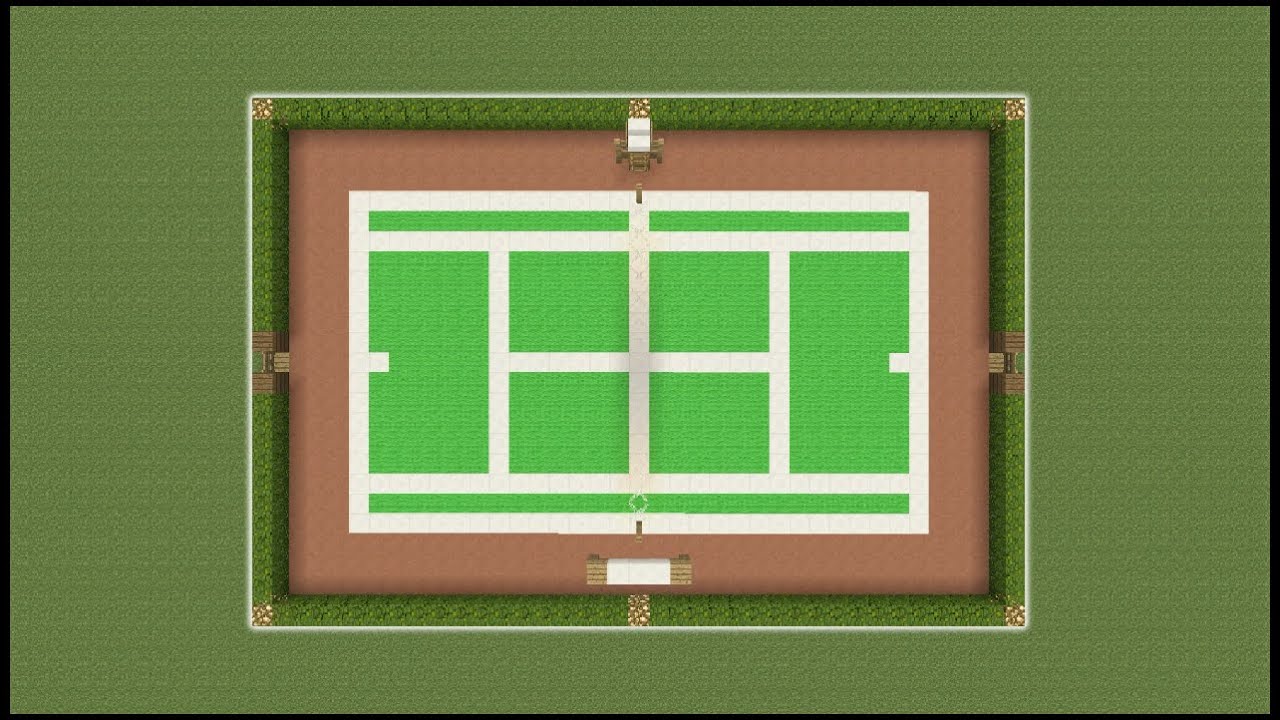This image is a detailed graphic rendering of a tennis or pickleball court, characterized by its precise and clean design. The overall composition features a vibrant green background framed by what seems to be a green hedge with gold corners. Within the main green border lies another rectangular green border, followed by a rusty or brown-colored frame. The central focus of the image is the white court itself, accentuated with sharp white lines demarcating various sections and boundaries of the court, including out-of-bounds areas for doubles and serving zones.

The court’s layout includes multiple shades of green filling the spaces between the white lines, creating a visually appealing contrast. The design includes four quadrants divided by the imaginary net area. It’s clear that this is not a photographic image but rather a high-quality computer-generated drawing, characterized by its sharp angles and clean finishes. The absence of a net and the empty court further emphasize the meticulously crafted graphic nature of the image, making it evident that it represents a sports field, most likely for tennis or pickleball.